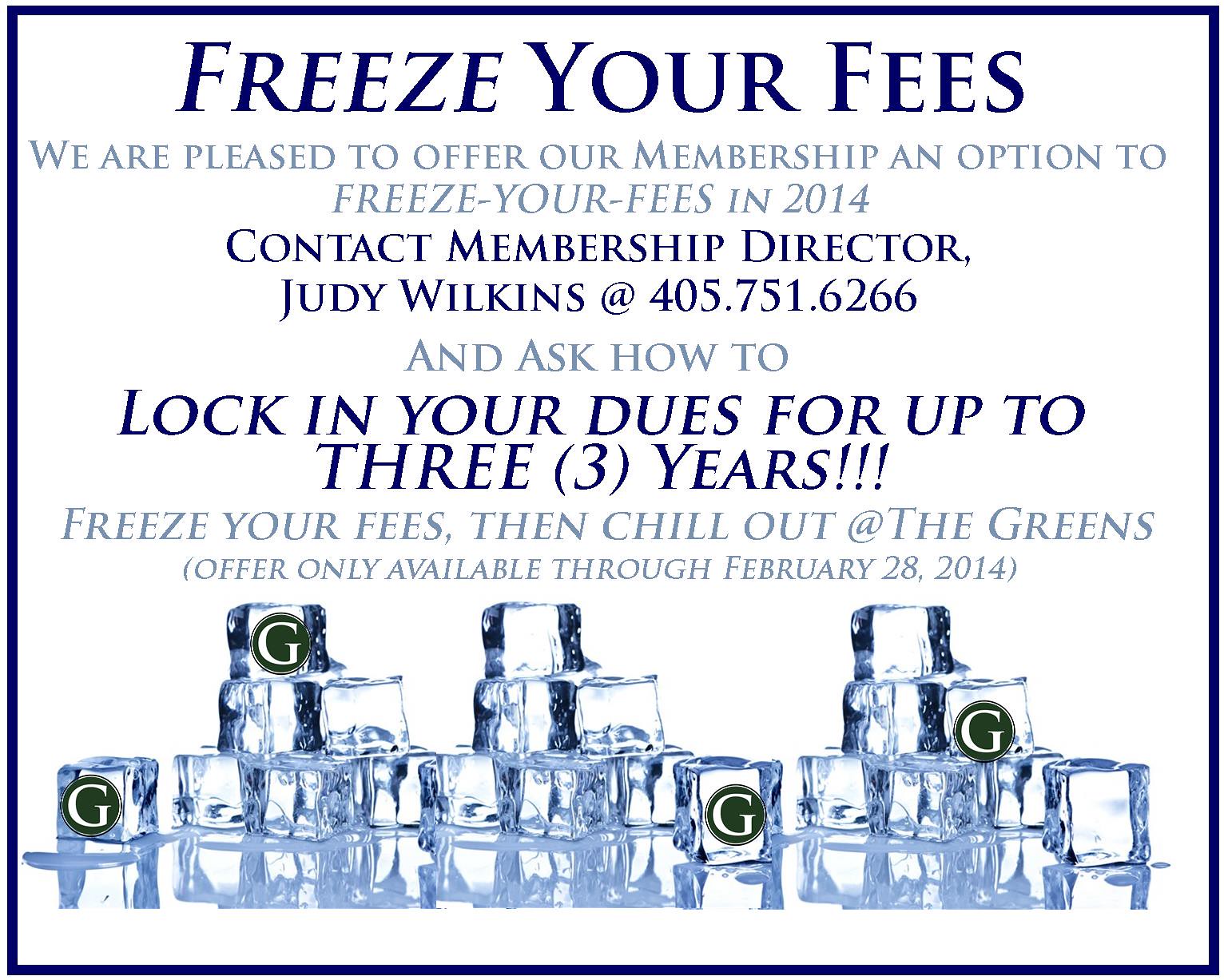The image is an advertisement poster titled "Freeze Your Fees" at the top in prominent black font. Beneath this, in gray font, it reads, "We are pleased to offer our membership an option to freeze your fees in 2014." The text then shifts back to black font, stating, "Contact membership director Judy Wilkins at 405-751-6266 and ask how to lock in your dues for up to three years." Following this in gray font, it says, "Freeze your fees then chill out at The Greens. Offer only available through February 28th, 2014." The bottom section of the poster features stacks of ice cubes, with four of the cubes displaying a white letter 'G' in a green circle. The overall color scheme and design elements give the poster a cohesive look, accentuated by a blue frame that complements the icy theme.